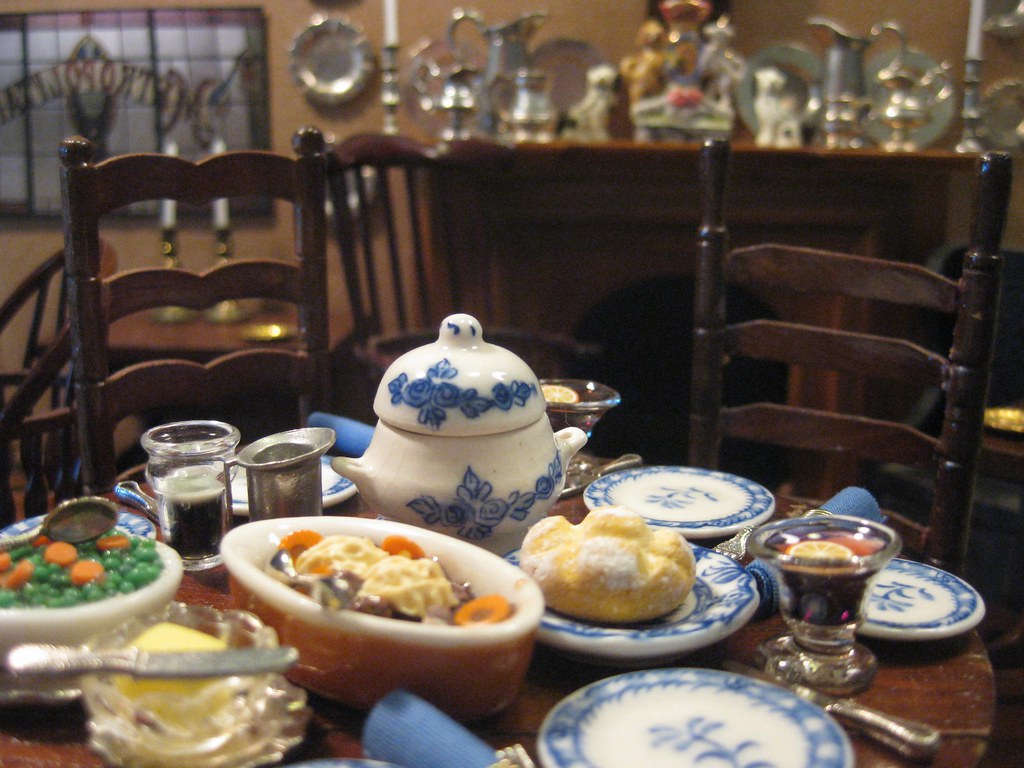The photograph depicts an elaborate dinner spread, likely a miniature setting given the plasticky and flat appearance of the items. At the bottom, a brown wooden-looking table is set with multiple blue-edged porcelain plates adorned with blue flowers, along with various dishes and platters at the center. 

One central white bowl, bordered with thin brown, contains mashed potatoes and carrots. To its left, a white bowl filled with peas and carrots features a resting spoon. Below these dishes, in the bottom left corner, a clear crystal container with a thick butter knife and a large yellow butter cube is positioned. 

Nearby, a large round loaf of yellow bread sits on one platter, while another dish holds fresh rolls. A ceramic teapot or sugar container, white with blue flowers, occupies a central spot. Adjacent are empty blue-edged plates and a goblet of brown liquid. The intricate table setting is completed with fine china and additional silverware, suggesting a formal or decorative occasion. 

In the background, an ornate wooden booth and an elaborate wooden chair allude to a restaurant-like atmosphere, enhancing the elegant yet miniature display.